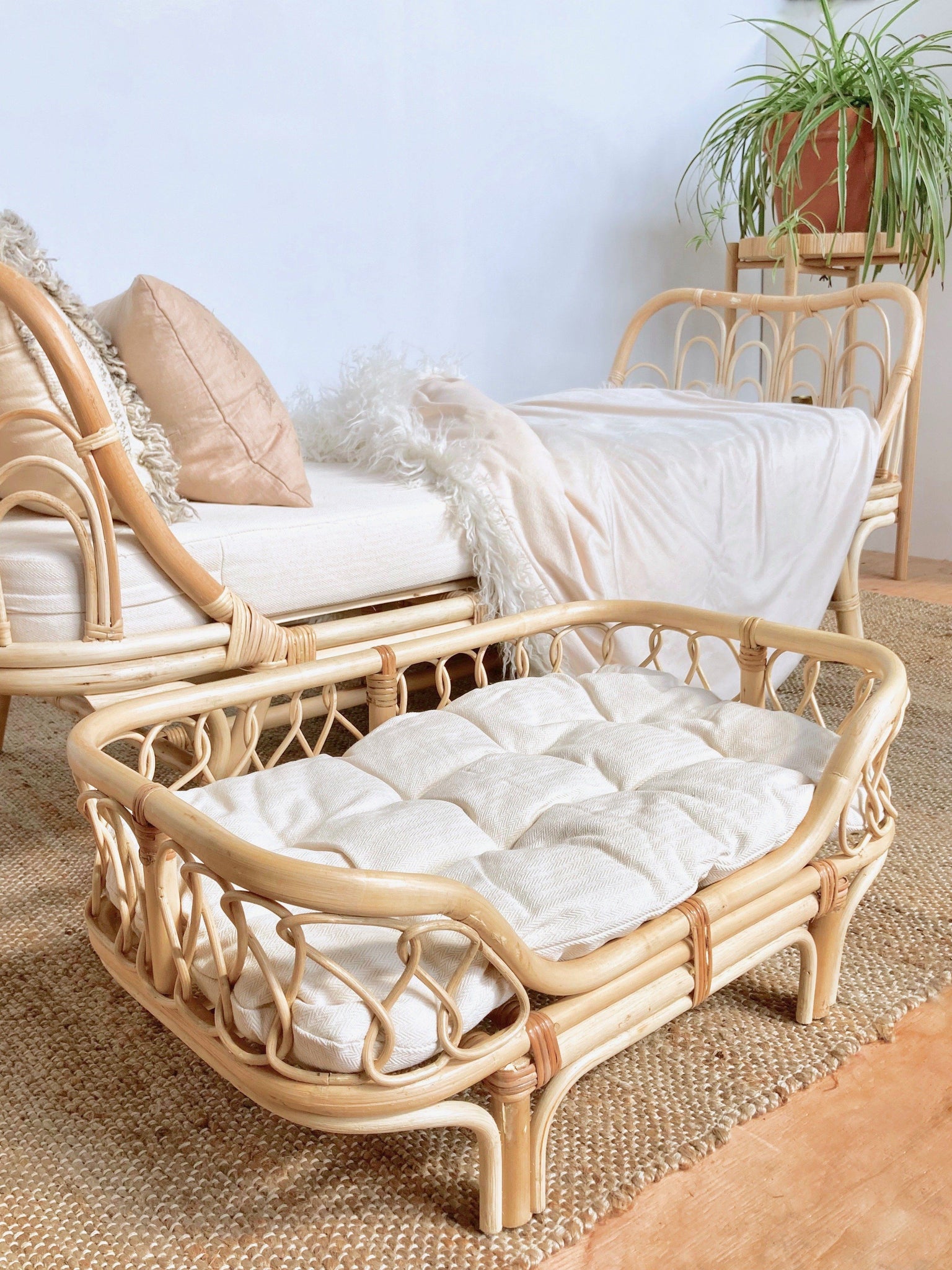This detailed color photograph captures a serene bedroom interior dominated by natural, earthy tones. The scene features a bedroom with white walls and showcases two main pieces of furniture: a daybed and an elevated pet bed, both constructed from a wicker-like material with wooden frames and intertwined, vine-like details. The daybed, set against a pale blue wall, is adorned with an unbleached cotton cushion, an ivory fringed throw, and two satiny accent pillows in varying shades of cream. On the floor, a woven jute rug with white accents complements the natural aesthetic.

Adjacent to the daybed is a uniquely crafted elevated pet bed with a similar wicker-style wooden frame and a quilted cushion. Both pieces rest on wooden laminate flooring with a cream-colored carpet beneath.

Adding a touch of greenery to the calm ambiance, a vibrant variegated spider plant sits in a terracotta pot atop a bamboo or light-colored wooden plant stand in the corner. This setting, though modern and minimalistic, exudes warmth through its use of natural materials and soft, neutral colors.